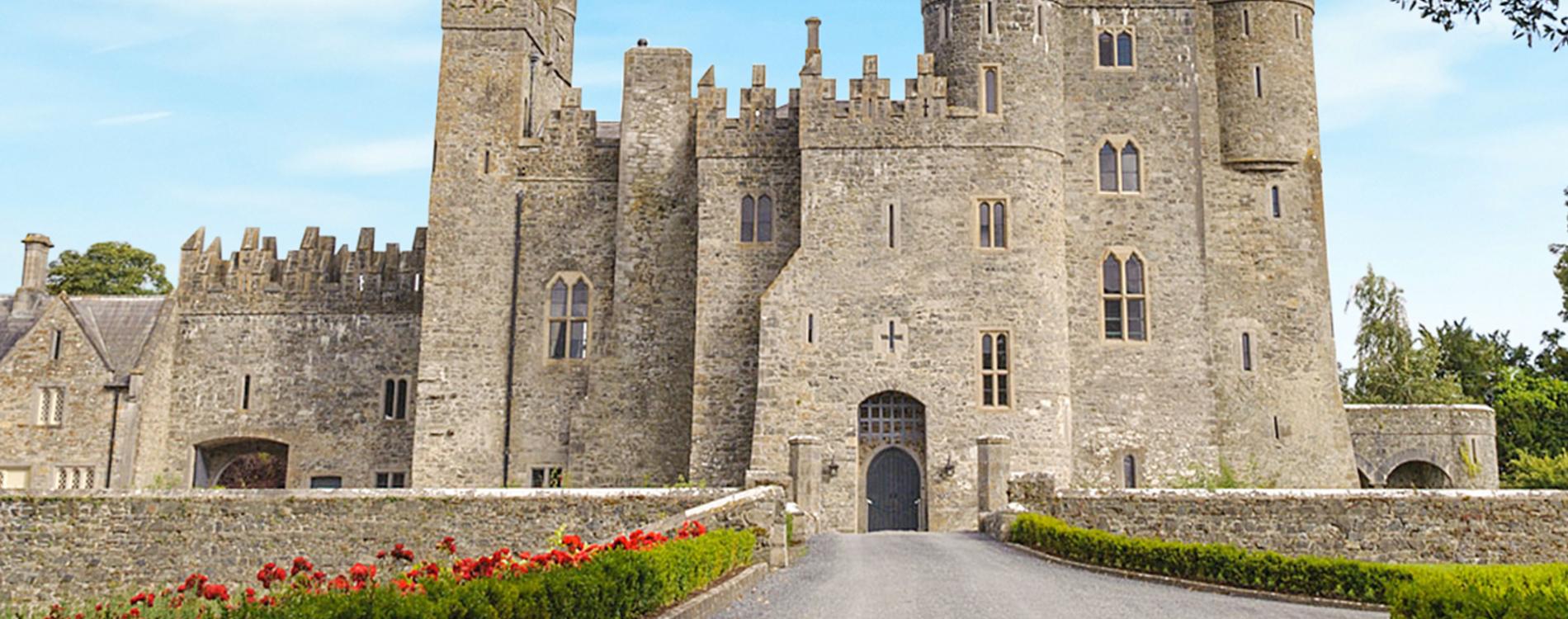This image captures the scenic entrance of a historic stone castle on a bright, lovely day with a clear blue sky dotted with a few clouds. The photographer is positioned on a paved walkway leading directly to the arched main entrance of the castle, which is accentuated by an iron grate that can be lowered for protection. This entrance features a distinct cross above the door. Flanking the walkway are low-cut hedges interspersed with vibrant red flowers, possibly poppies, and green shrubs. The castle, made of light-colored stone, is remarkably well-preserved given its age. It features narrow windows and turrets, indicative of its medieval design, and likely served defensive purposes with positions for archers or gunners. The structure rises several stories high on the right, each floor showcasing pairs of arched windows. Surrounding the castle are lush green trees, enhancing the picturesque and tranquil atmosphere.